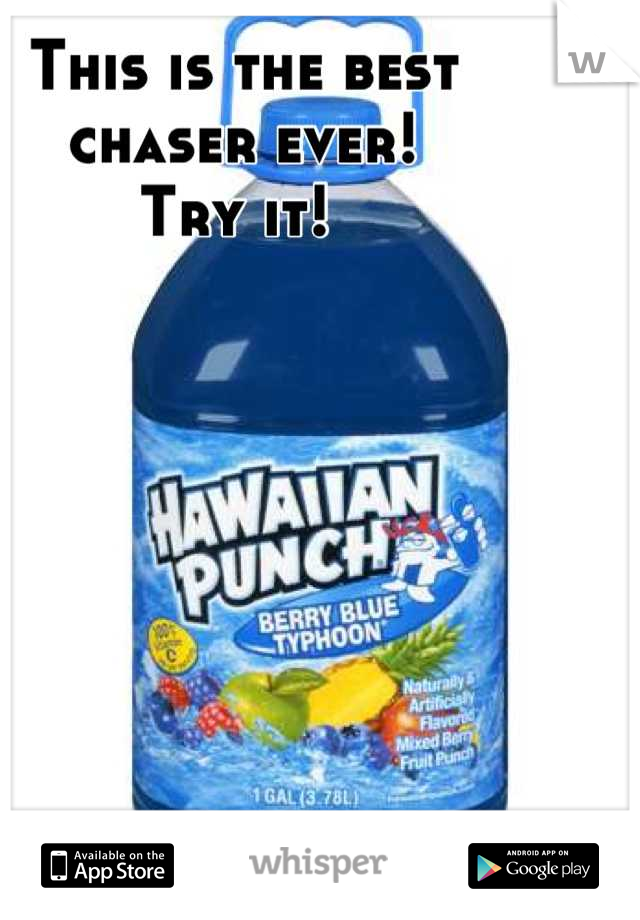The image is an advertisement for Hawaiian Punch Berry Blue Typhoon, set against a completely white background. Prominently displayed is a large, 1-gallon (3.78 liters) bottle of the blue mixed-berry fruit punch, labeled as naturally and artificially flavored, offering 100% of the daily recommended value of vitamin C. The label features a character with red hair surfing on a snowboard amidst a splash of water, surrounded by illustrations of various fruits including pineapple, green apple, blue raspberry, red raspberry, blueberry, and red apple. Across the top of the image, bold black text declares, "This is the best chaser ever! Try it!" In the bottom corners, icons indicate the app's availability on the App Store and Google Play with the word "Whisper" in between. The top right of the image features a letter "W," which is part of the Whisper platform logo advertised in the image.